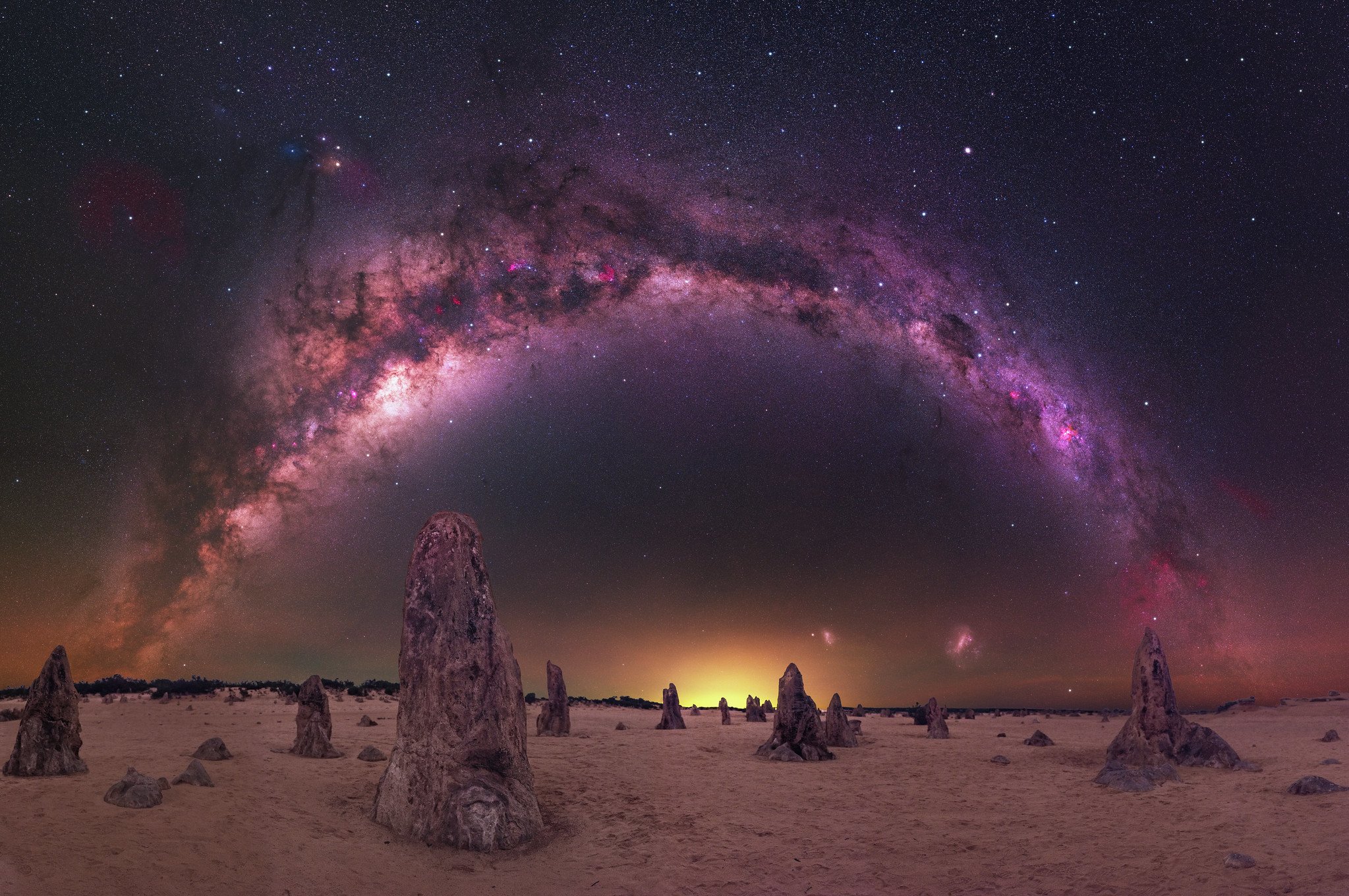The photograph captures a stunning desert landscape at night. The ground is covered in light tan sand, dotted with medium-sized, skinny rock formations that protrude prominently, resembling small reddish clay mountains. The horizon glows with a faint yellow light, likely from the setting or rising sun. The night sky above is a mesmerizing mix of purples and pinks, highlighted by a striking, rainbow-shaped cloud formation that hints at a galaxy. This celestial display, possibly achieved through long exposure photography, showcases vivid nebulae, bright and dark patches, and countless stars scattered throughout the sky. The overall scene exudes an ethereal beauty with its cool, dark purple tones and star-studded galactic spectacle.